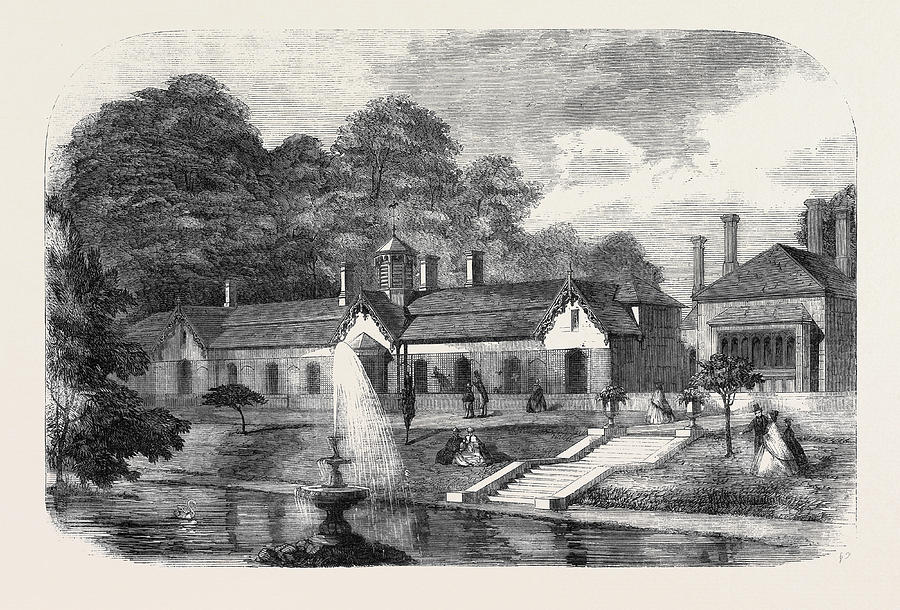The image is a detailed black-and-white drawing, likely made with graphite or pen, set against a peach-colored background. At the front and center of the drawing is a fountain shaped like a birdbath, with water spouting from the top. To the left of the fountain, there are several tall trees and a large building with a sloped roof featuring three peaks, numerous doors, and windows. Moving to the right, a set of stairs descends from a sidewalk area where people are seen walking towards a smaller building that resembles a shed with four chimneys. People are also seated on a nearby lawn. On the right side of the drawing is another building with columns and arched windows, partially obscured by the foliage. In the lower right corner, a body of water extends across the bottom of the image, possibly a pond or small river. This idyllic scene includes various natural elements, such as clouds and additional small trees scattered throughout the background, lending a serene, detailed ambiance to the artwork.